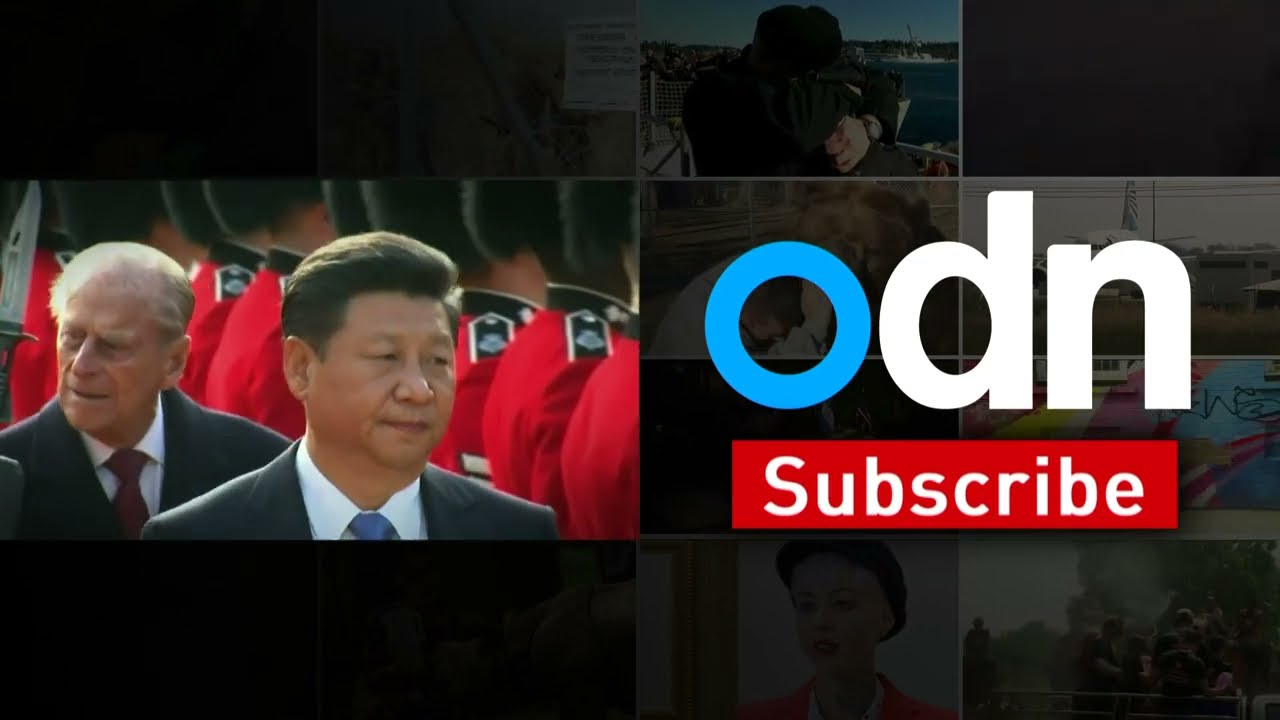The image captures a vibrant outdoor scene during the daytime, showcasing a massive rally in Washington D.C. In the center of the image, there is a large crowd of over 500,000 people, predominantly women of various ages and all of Caucasian descent, as indicated by their visible attire. They are marching and holding signs, many of them wearing distinctive pink pussy hats. The participants are donning coats, hinting at a cooler season, and are surrounded by leafless trees.

Above the crowd, the imposing architecture of government buildings, including what appears to be the Capitol building, serves as a backdrop. The Capitol's facade features multiple American flags draped from its pillars, adding to the patriotic atmosphere. The white dome of the Capitol, topped with a statue, is prominently visible, partially shrouded by a light gray, cloudy sky.

At the bottom of the image, a transparent black banner running from left to right displays white text that reads: "The largest rally was in Washington D.C. where crowds numbered more than 500,000." Specific words like "largest rally," "Washington D.C.," "crowds," and "more than 500,000" are highlighted in bold, emphasizing the magnitude of the event. This combination of visual and textual elements suggests the image might be part of an informative slide, perhaps from a TV show or documentary.